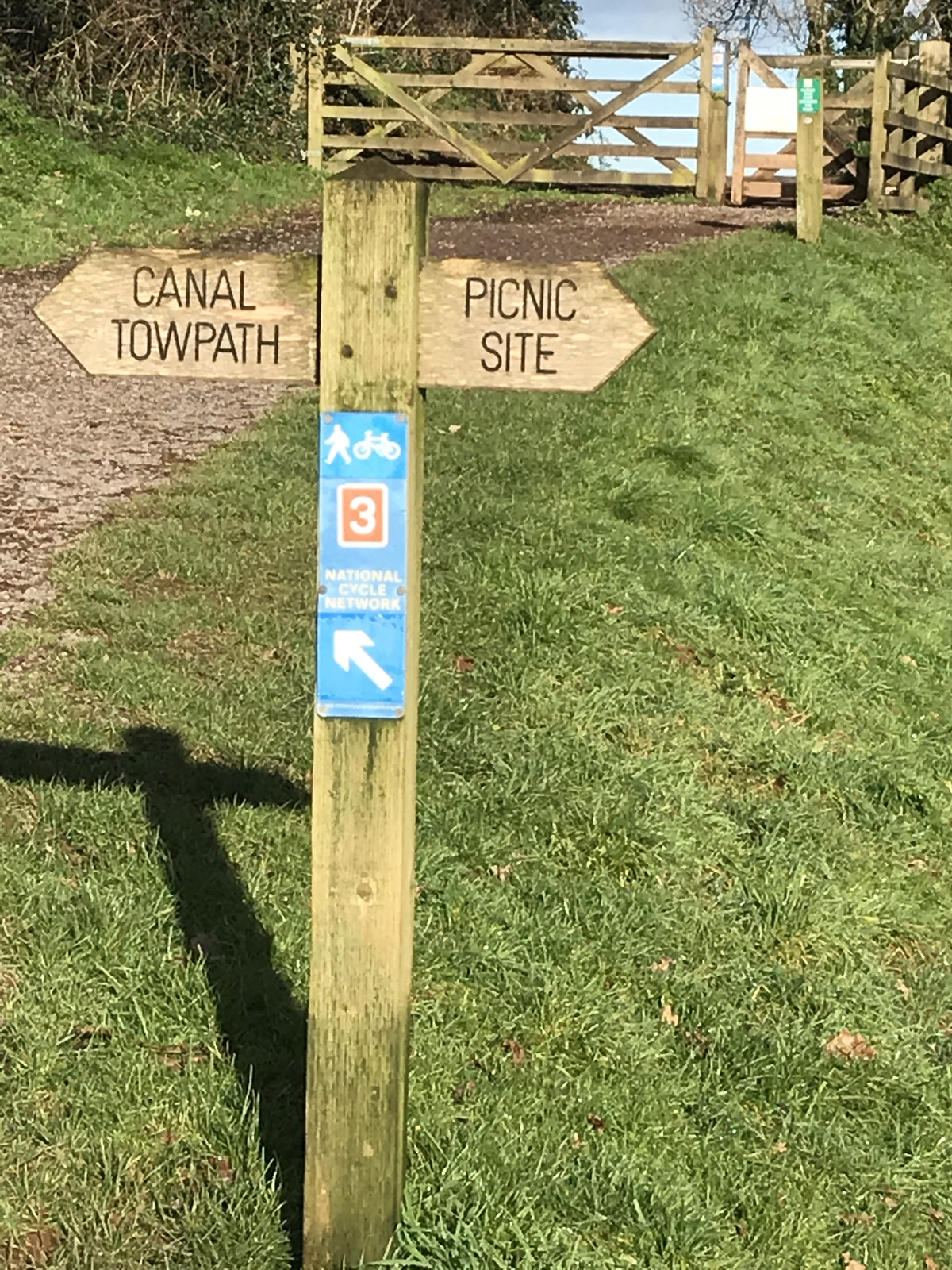The image depicts a tall, rectangular wooden signpost firmly placed in a grassy area, slightly left of the photo's center. To the left of the signpost lies a dirt and stone path that winds up towards a closed wooden gate in the background. Adjacent to the gate is another post with a green sign, potentially indicating an area for hikers. The main signpost in the foreground features two wooden arrows: the left arrow pointing towards the "Canal Towpath" and the right arrow indicating the "Picnic Site." Additionally, attached to the signpost is a blue sign featuring a white silhouette of a hiker and a biker, with a diagonal arrow pointing left. Below this image, a red square with a white number "3" denotes the National Cycle Network. Apart from the sign, the scene also includes grass, some brush, and an absence of people or bicycles, with a serene horizon marked by a wooden fence and sky.